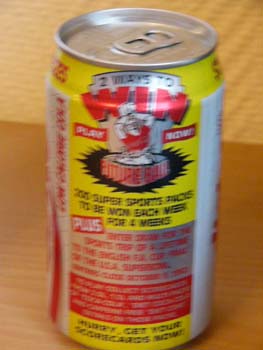A slightly blurry photograph captures the backside of a can, likely Diet Coke, resting on a light blonde wooden table. The top of the can is silver, while the main body features a mix of silver, red, and yellow backgrounds. Prominently displayed on the can is a message with the words "Two Ways to Win" and "Play Now," accompanied by a small graphic figure in the center. Below this, black text appears but is difficult to decipher due to the blurriness. Further down the can, a silver section with red text also proves challenging to read. This is followed by a red section with silver text that is almost entirely illegible. At the bottom, a yellow rectangle with black text is similarly hard to distinguish. The intricate details of the can's promotional design elements are obscured by the photograph's lack of sharpness.